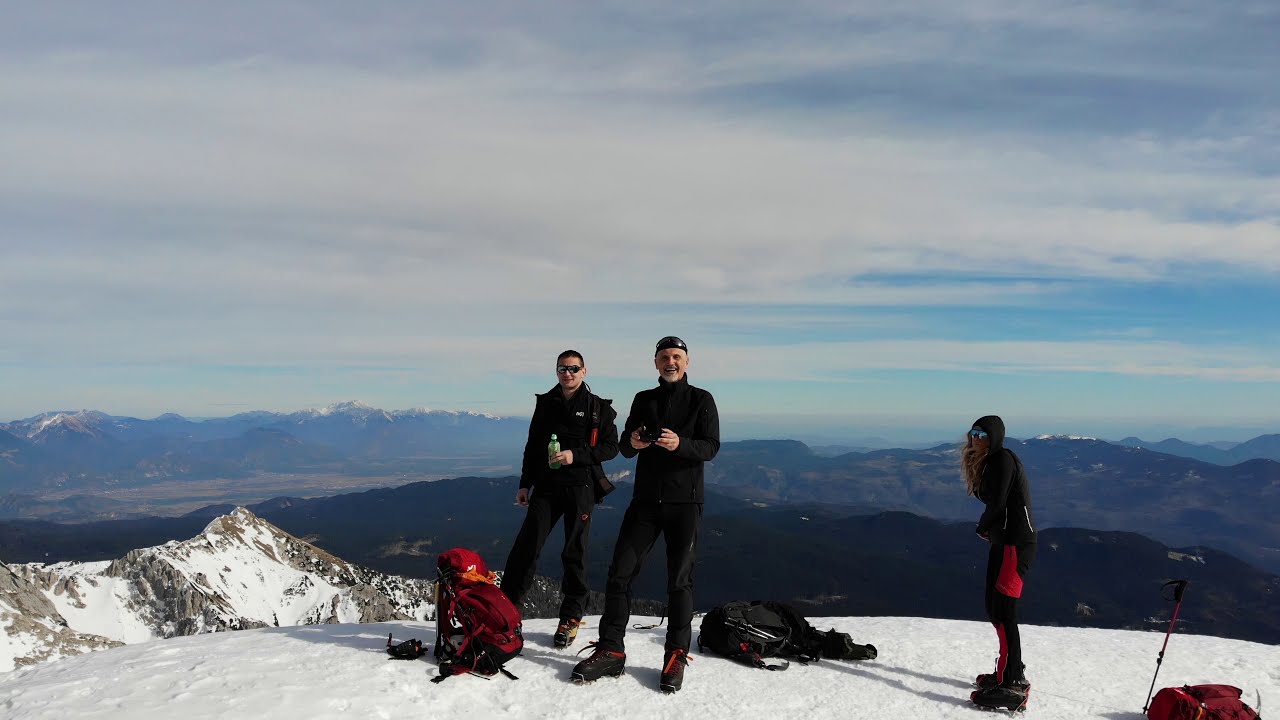The image captures a high-altitude moment where three hikers stand triumphantly atop a snow-covered mountain peak, likely at the end of a strenuous hike. Clad in black long-sleeve jackets and heavy-duty snow pants, the trio appears well-prepared for the freezing conditions. Their black ski boots further emphasize the rugged, cold environment. The group composition includes two men on the left and a woman on the right, who has long hair cascading down and wears a black hood over her head, with black and red accents on her outfit. The central figure of the man smiles directly at the camera, while the woman on the right glances back over her left shoulder. Scattered around them on the snow are multiple backpacks, including a red one on the left, a black one on the right, and another red one in the bottom right corner, accompanied by a red ski pole. The expansive background features a vast mountain range stretching out to the horizon under a mostly cloudy sky, with light blue patches peeking through.